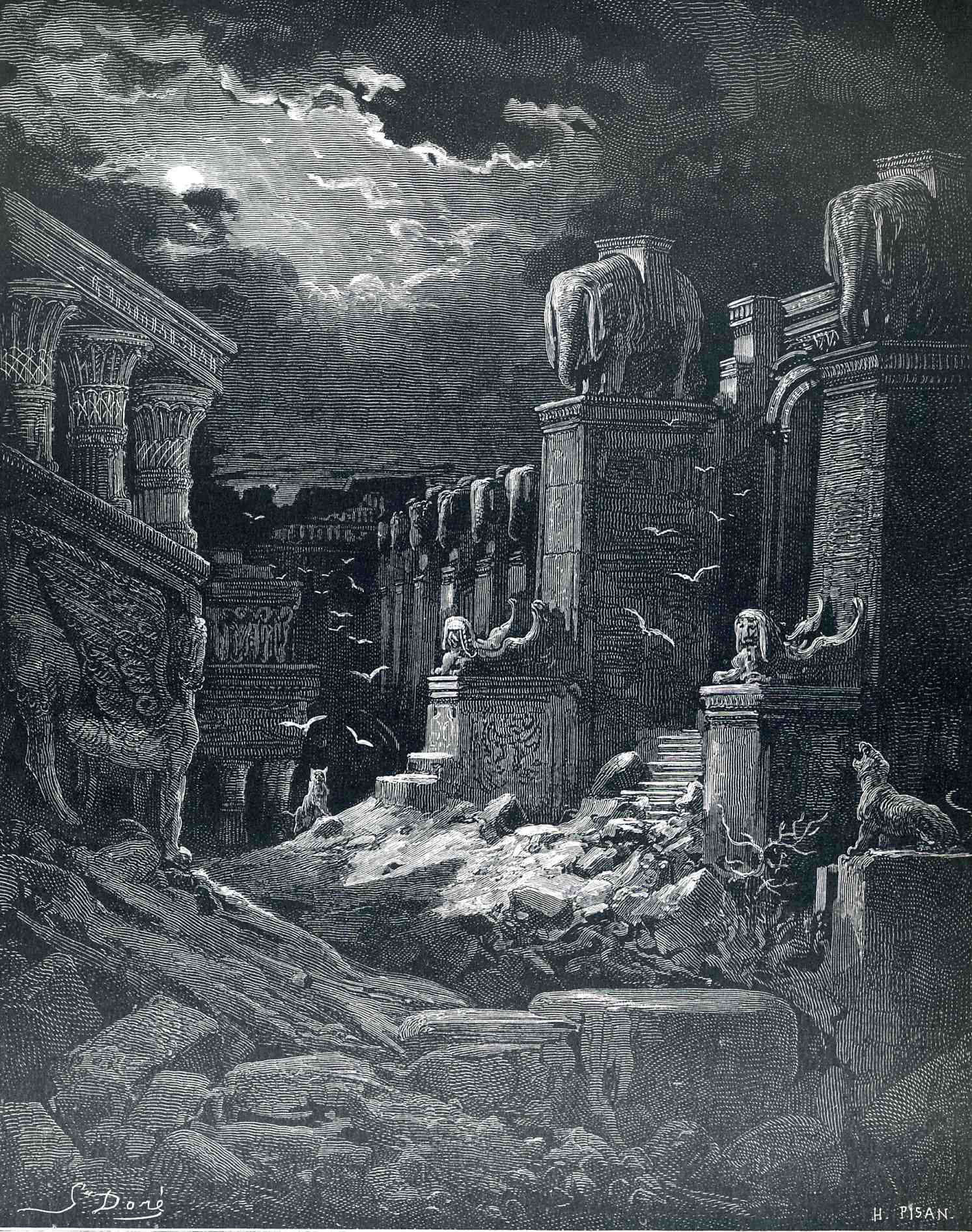This grayscale pen and ink drawing depicts a nighttime scene of ancient ruins, showcasing intricate hatching and cross-hatching techniques. The foreground features a grand entranceway flanked by large, crumbling pillars, each topped with statues of elephants. At the base of the stairway between the pillars, rocks and debris are scattered, hinting at the structure's dilapidated state. On either side of the stairway are statues of unidentified animals, adding to the mysterious ambiance. To the right of the scene, a sculpted tiger keeps a silent watch. The sky is heavily clouded, with the moon faintly visible through the breaks in the clouds, casting a subdued glow over the entire scene. Birds are seen flying around the ruins, enhancing the sense of abandonment and decay. Handwritten in white ink, the initials "S done" appear in the bottom left corner, while "H Pisan" is inscribed in the bottom right, possibly indicating the artists involved.